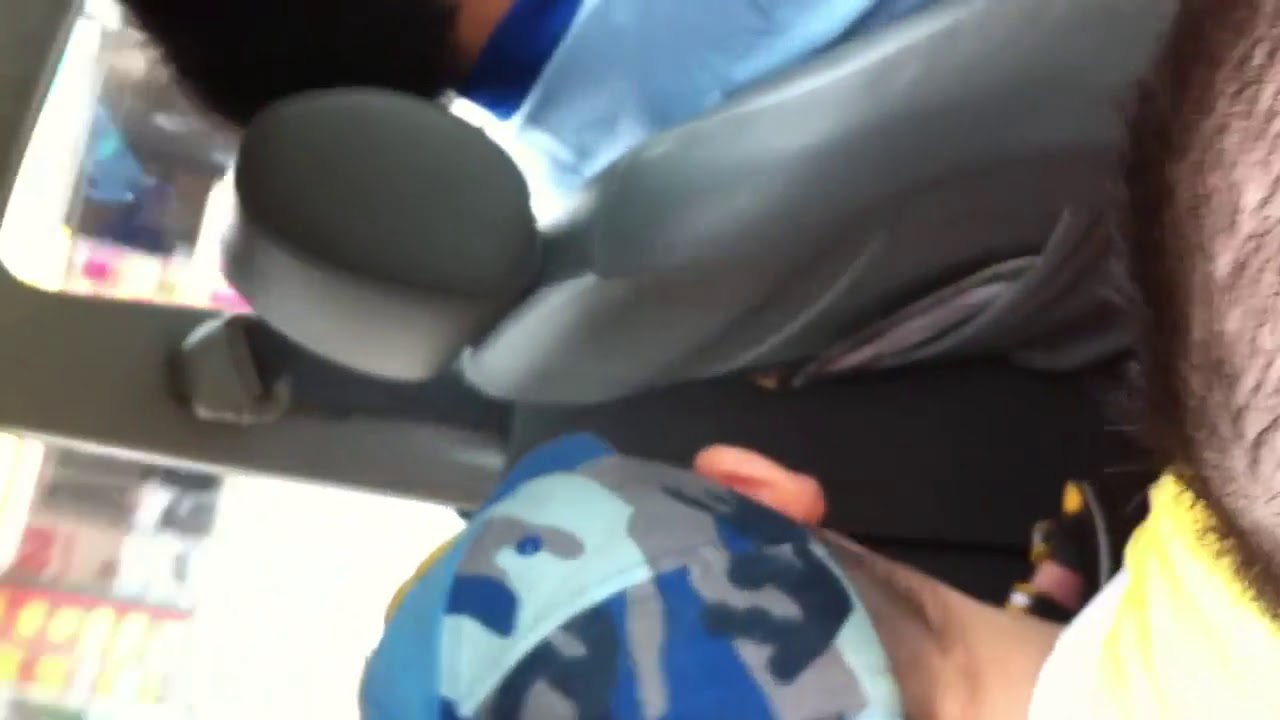This detailed, descriptive caption combines elements from each contributor, emphasizing shared and repeated details:

This image, although rotated 90 degrees to the left, provides a close-up view of the interior of a vehicle, likely a bus due to visible windows and seating arrangements. At the bottom of the image, the back of a person's head is visible, wearing a blue camouflage hat with a dark blue bill. In front of this individual is another passenger seated, who is dressed in a light blue t-shirt with a dark blue collar. This second passenger has dark hair that appears either very short or possibly balding. The image is brightly lit, indicating daytime, and features the vehicle's gray seats. The surroundings outside the windows are blurred, but hints of a storefront with signs are discernible. The overall scene suggests a group of individuals traveling, with no faces visible, only the backs of their heads, emphasizing the anonymity of the travelers.